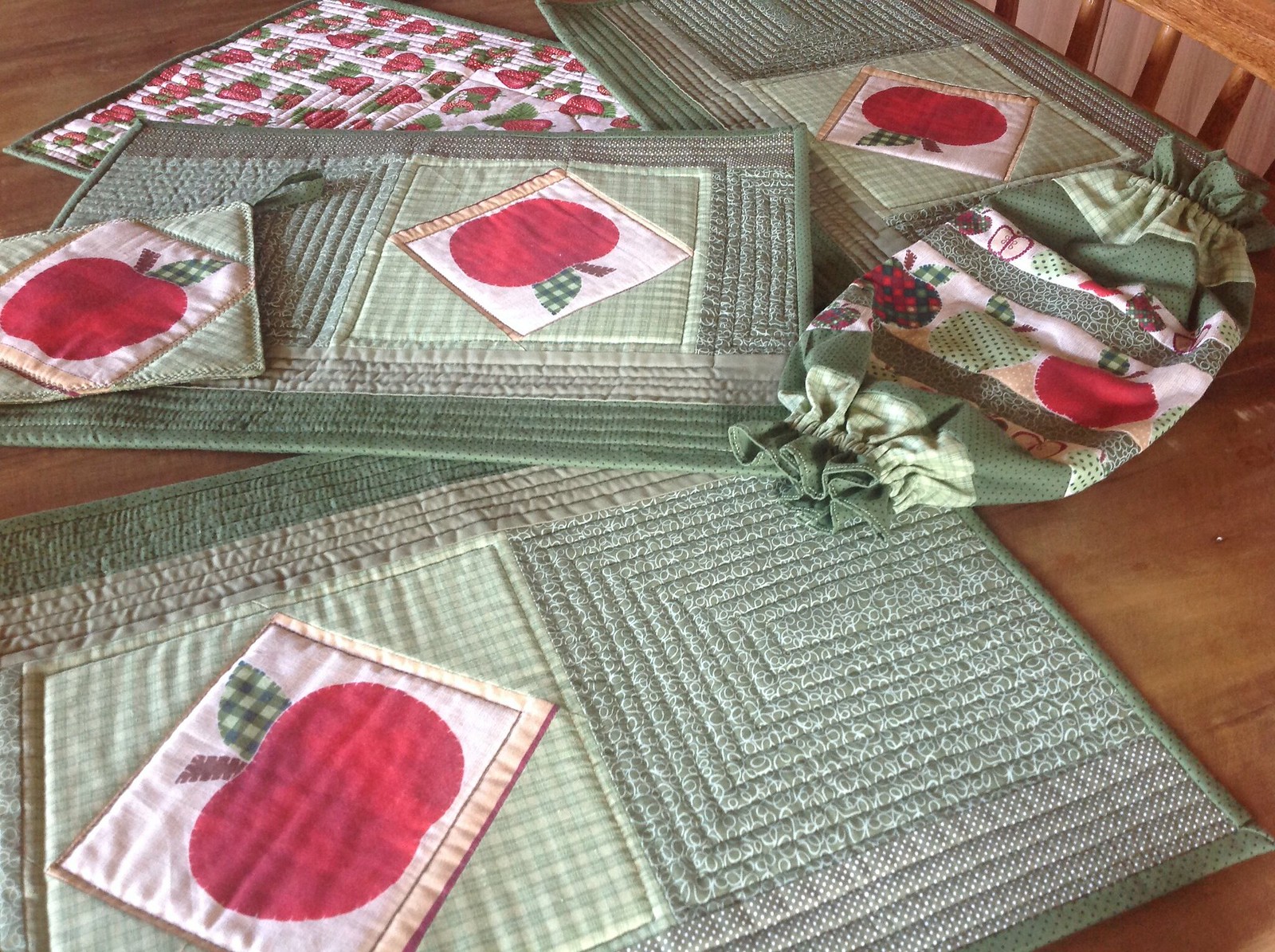On a light-colored wooden dining or kitchen table, there's an arrangement of ornately quilted table decorations. The set features three placemats, an oven heat pad, a small towel, and a fruit-shaped bag holder, making a total of six pieces. Each item prominently displays a red apple with a brown stem and a green checkerboard leaf, which is the main motif. 

The placemats are detailed with a diagonal apple on the left side, bordered with strips of light and dark green quilted fabric, and a calico green pattern on the right. One of the placemats includes white squares filled with red apples and green checkerboard leaves. A peek beneath the placemats reveals another mat, possibly a trivet, characterized by a similar apple design and a green border.

The topmost object is a potholder, matching the apple motif and featuring a green loop for hanging, positioned diagonally. The final piece is a tubular bag holder with scalloped, elasticized edges, crafted from the same apple-themed fabric, intended for storing plastic bags. In the background, a wooden chair or bench made of slats is partially visible, adding to the cozy and rustic ambiance of the setting.